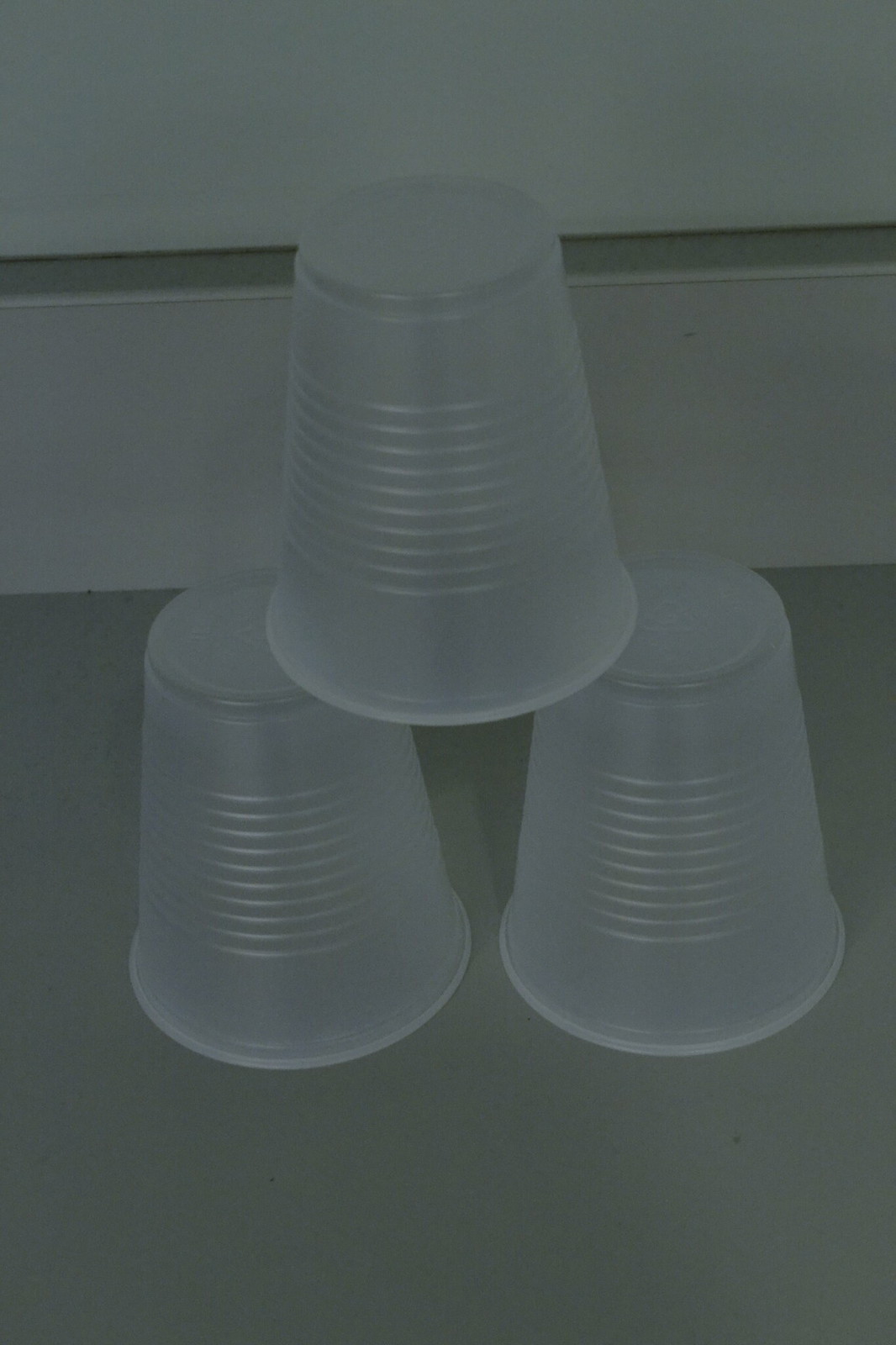This indoor, close-up photograph showcases three clear plastic cups, each about eight or nine ounces, stacked in a pyramid formation—two at the bottom and one on top. The cups, which are brand new and unused, feature horizontal ribbing along their midsections and are devoid of any coloring or printed text. Positioned on a white table with a pale backdrop, the overall image is rather dark and somewhat grainy, although it remains in focus. A faintly tan horizontal line appears on the wall in the background, suggesting a division or seam in the surface. The cups, translucent and colorless, resemble the style typically found at picnics or doctor's offices. The photograph is taken from above at approximately a 45-degree angle, tightly framing the subjects to emphasize their reflective ribbed texture.